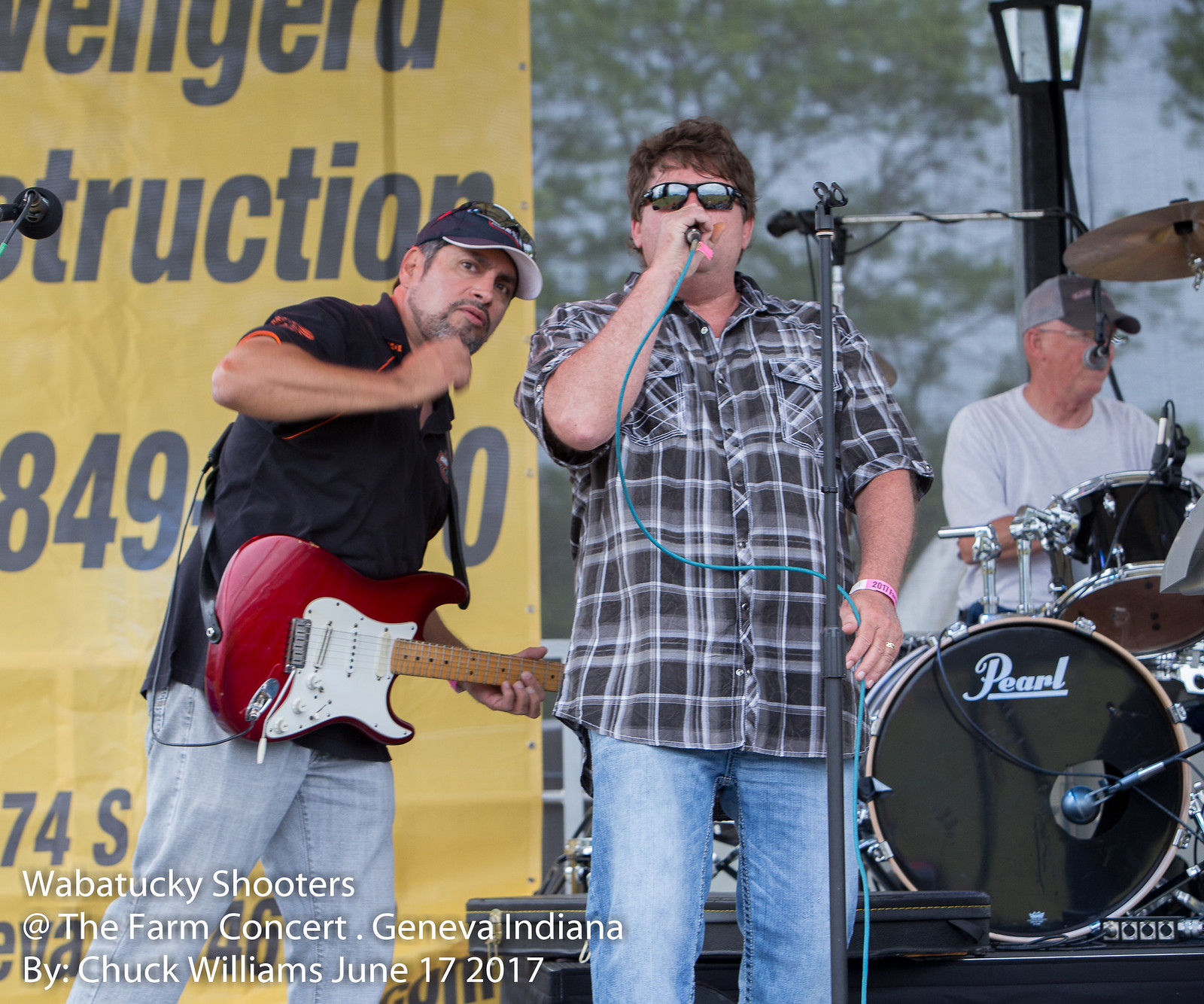This image captures an outdoor concert set against a park backdrop with light blue skies and trees. On the right side, an older drummer, possibly in his 50s, sits behind a black Pearl drum kit, identifiable by the white "Pearl" label on the front drum. He wears a gray cap, wire-framed glasses, and a white t-shirt, with a microphone placed in front of him, suggesting he may also sing. In the image's center, the lead singer, wearing a short-sleeved plaid brown and white shirt, blue jeans, and sunglasses, clutches a microphone with a blue cord that partially obscures his face. Next to him, a guitarist, dressed in a black shirt with orange accents, light jeans, and a baseball cap, leans slightly towards the singer. His guitar, resembling a Stratocaster, features a red body with a white pickguard. Behind the band members, a yellow banner with "something construction" and a phone number is visible, along with a black streetlight nearby. In the image’s bottom right corner, a watermark reads, "Wabatuckee Shooters at the Farm Concert, Geneva, Indiana by Chuck Williams, June 17, 2017."